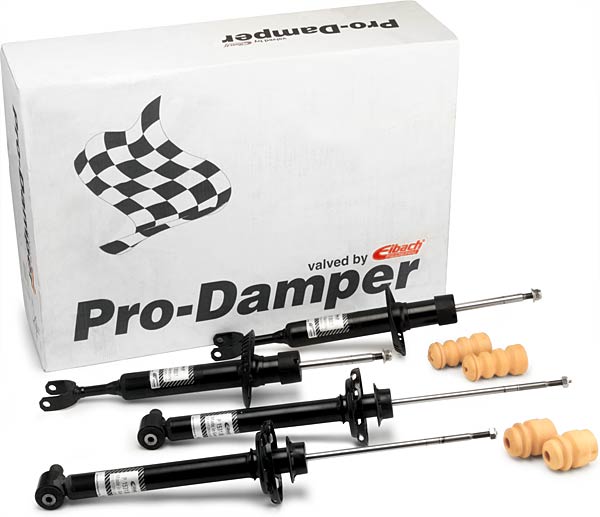The image features a white box with a black and white checkered flag design on it, positioned slant-wise in the top left corner against a white background. The box bears text that reads "Pro Damper" at the bottom and "Valved by Eibach" above it in smaller red letters with a logo. In front of the box lie four black-handled metal poles placed sideways, each with narrow metal tips. To the right of these poles are several brown cork pieces. The color palette includes black, white, red, silver, and brown. This setup could be used in a tool store display, an online presentation, or on a home improvement website.